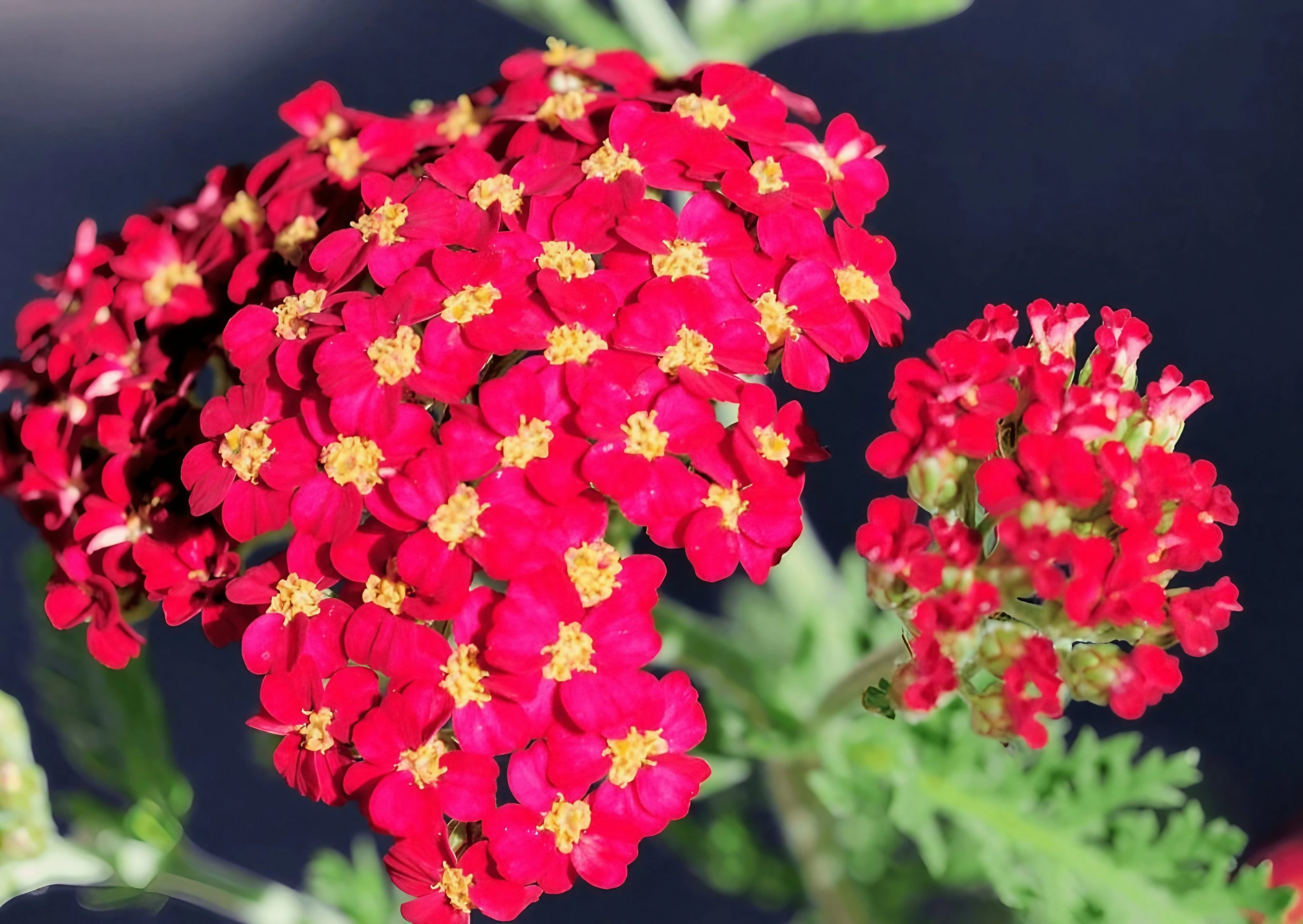This close-up image showcases a vivid display of bright red flowers with star-shaped yellow centers, set against a dark, indistinct background of blue and black hues. The flowers in the foreground are in sharp focus, with intricate details visible on each petal, while the greenery of the plant, including leaves and stems, appears blurred. The composition consists of two distinct clusters of blossoms: a larger, densely packed section on the left and a smaller but equally vibrant cluster on the right. The petals of the flowers are numerous and trumpet-shaped, prominently highlighting their bright red color punctuated by yellow star-shaped centers. As the flowers recede into the background, they become progressively blurry, emphasizing the contrast between the detailed foreground and the hazy, unfocused backdrop.